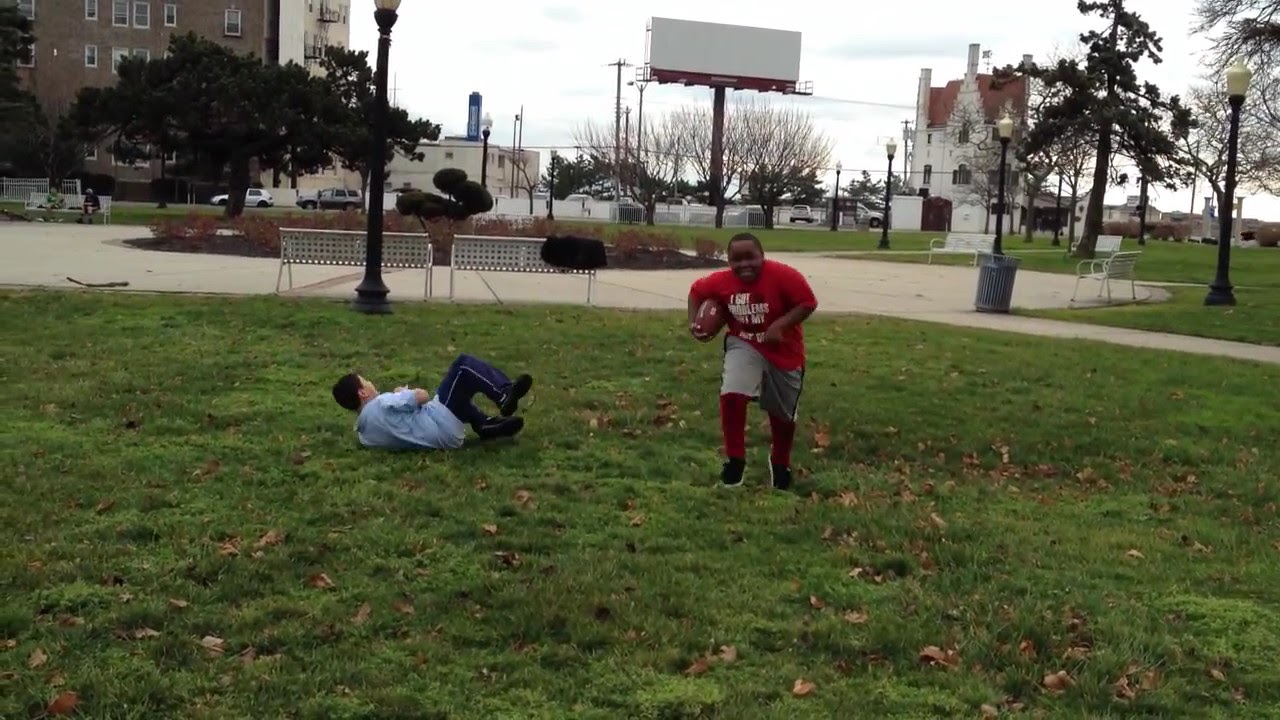The image captures a lively scene in a park where two young boys are playing football. The focal point of the scene is a small African American boy in a red t-shirt with white text, holding a brown football under his right arm while running toward the camera. He wears grey shorts over red leggings and black shoes. On the left side of the image, a young boy with short black hair, possibly Caucasian, lies on the grass after an apparent tackle attempt. This boy is dressed in a light blue shirt, dark blue track pants, and black shoes. The grassy field is scattered with brown leaves, and in the background, there are various park elements, including a central median with plants, black metal light poles, benches, and garbage bins. The park area is framed by sidewalks and features buildings, houses, and cars in the distance. The sky above is partly cloudy with patches of blue, adding to the dynamic ambiance of this park scene.